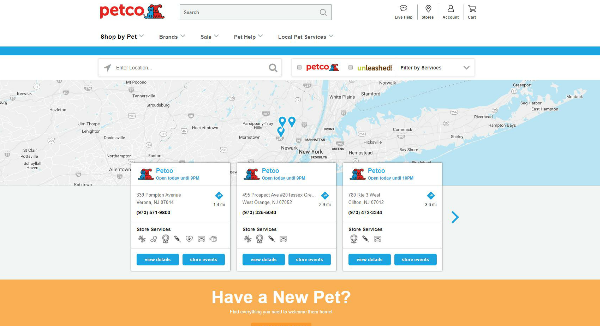The image is a landscape-format screenshot of the Petco website, as displayed on a laptop. The website's branding is prominently featured with the "Petco" logo in the top left corner, written in lowercase red letters. Adjacent to the logo is a charming cartoon illustration showing a blue cat snuggling next to a red dog. 

At the top of the webpage, there are multiple navigation tabs, including options such as "Shop by Pet" and "Branch," though some are unreadable due to pixelation. The "Shop by Pet" tab is currently selected. 

Below these tabs, the main content of the screen includes a map interface, resembling a Google Map, indicating various Petco locations within the New York and New Jersey area. Three specific Petco offices are highlighted, each accompanied by their respective addresses and contact information.